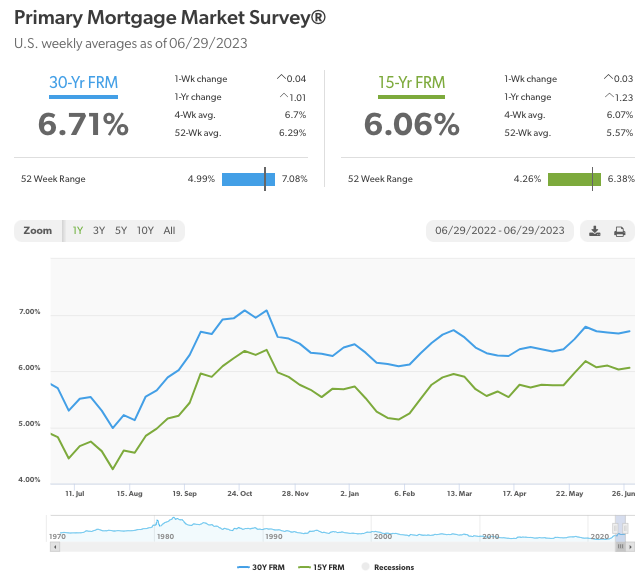The image is a detailed screenshot from a financial website, specifically focusing on mortgage rates. The top part of the image has a clean white background with a prominent black text header that reads "Primary Mortgage Market Survey®". Directly beneath this, there is a subheading that states "U.S. weekly averages as of 06/29/2023".

The central focus of the image is the updated mortgage rates, displayed prominently in larger text: "30-year FRM, 6.71%" and "15-year FRM, 6.06%" with the latter highlighted in green. Next to these figures, detailed information is presented, encompassing metrics such as "One week change," "One year change," "Four-week average," and "52-week average."

The lower section of the image features a bar graph spanning the width of the frame. This graph includes a blue line representing the 30-year fixed-rate mortgage (FRM) and a green line representing the 15-year FRM. These lines undulate similarly to an EKG chart, illustrating the fluctuations in mortgage rates over specific periods.

Overall, the image provides a comprehensive snapshot of current and historical mortgage rate data, helping viewers quickly interpret trends and changes in the market.